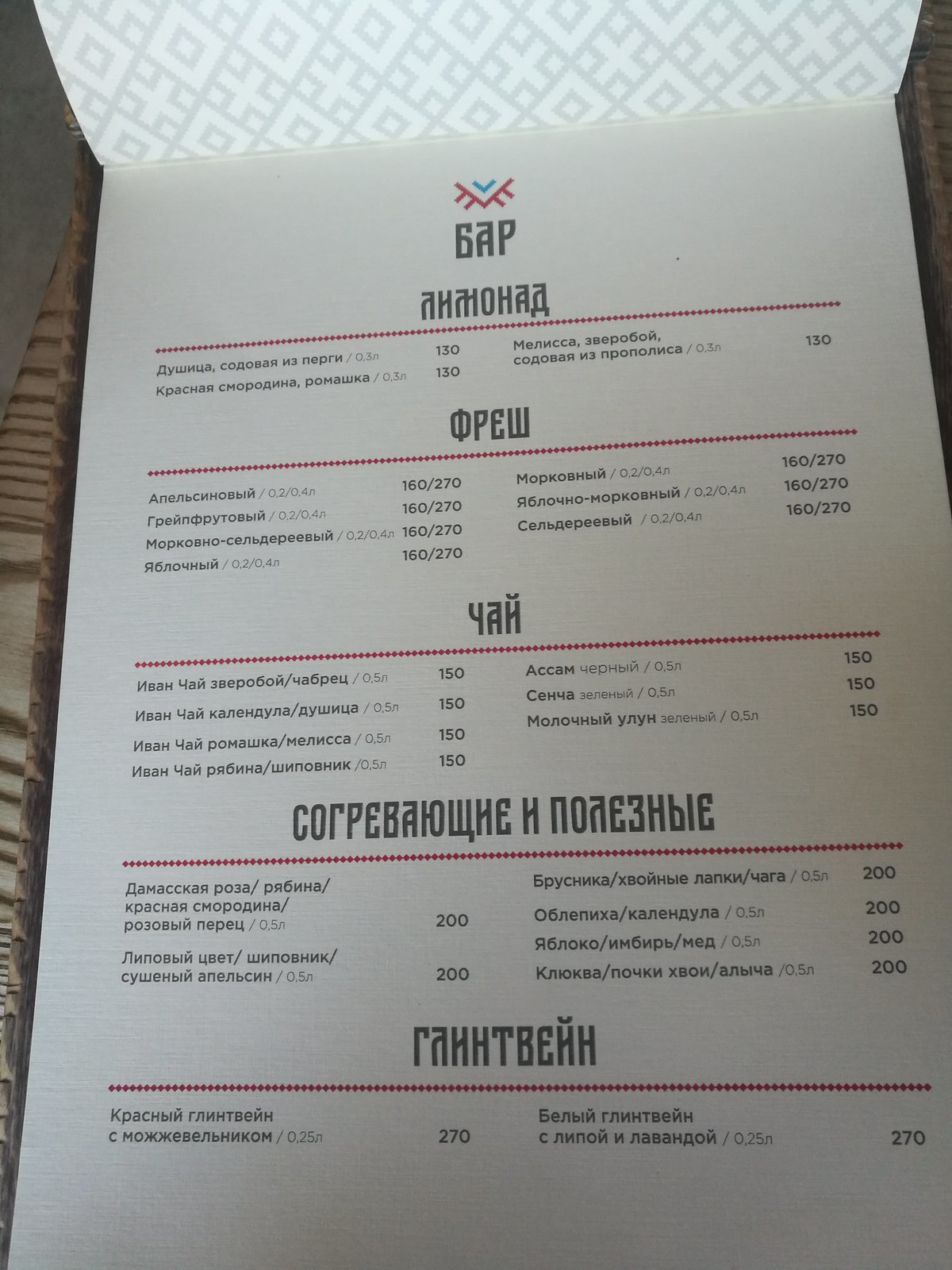The image depicts a close-up view of what appears to be a Russian menu or price list. The document is positioned against a grey-toned cover, featuring an alternating diamond and cross-X pattern, reminiscent of a notebook or menu holder. This cover is partially open, revealing the main page.

At the top of the menu, there is a simple logo rendered in red and blue. Beneath the logo, the menu text is divided into five distinct sections, each introduced by a header. These headers are underlined with red dotted lines. Within each section, items are listed alongside numbers, which likely represent prices. Some entries display two numbers separated by a backslash, potentially indicating different sizes or varieties of the items listed. The menu is placed on a wooden surface, visible at the top right and left edges of the image, suggesting that it is laid out on a table or similar flat surface.